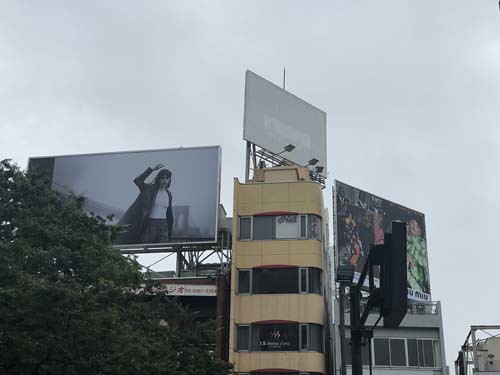The rectangular photograph captures a daytime outdoor scene dominated by a three-story yellow building with large, glass windows on each floor, framed in thin silver. The building, which reflects a slightly dated modern architectural style, could be from the 1970s or 1980s. Each window features a large central pane flanked by two narrower side panels. This yellow structure seems to be part of a cluster of buildings, as different architectural styles and colors are visible on either side. Atop the yellow building is a skewed billboard angling down and to the right, its faded white text rendered illegible. Perpendicular to this billboard is another, showing a woman with shoulder-length dark hair, raising her right arm and dressed in a white shirt over dark pants against a gray backdrop – possibly a black and white advertisement reminiscent of high fashion or luxury brands. Below and to the left of the building, a lush green tree occupies a portion of the frame, adding a touch of nature to the urban setting. The top right section includes another billboard partially covered by a structure resembling a basketball hoop in profile, showing people in bright clothing, although the image details remain unclear. The cloudy sky forms a muted backdrop to the scene, lending a tranquil and overcast ambiance.